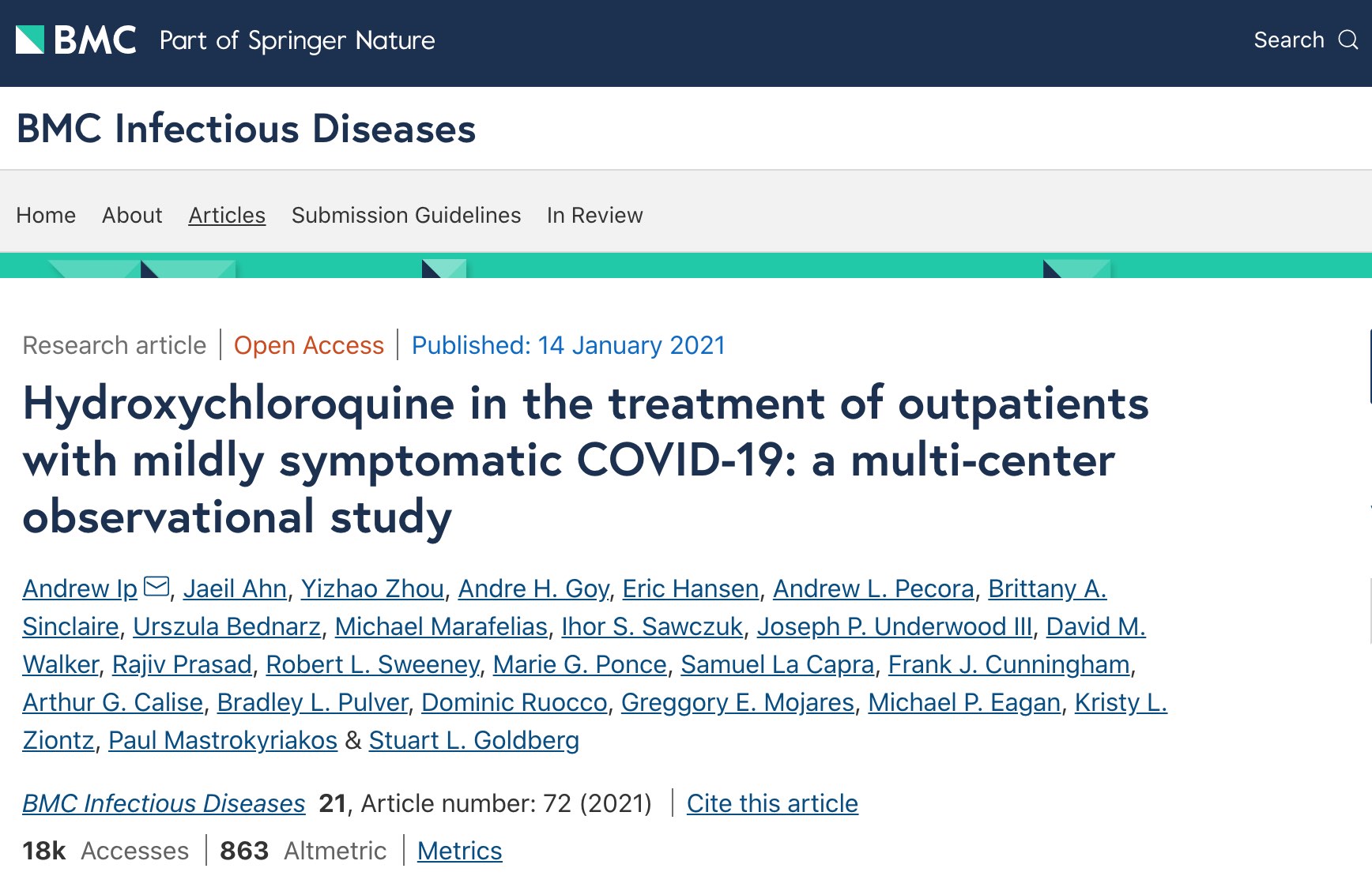This is an image from a news website, showcasing a detailed layout of an academic article. The top part of the image features a dark blue border. On the left side, there is a square with the top left corner down to the bottom right corner in white, and the top right portion in a teal color. Inside this square, "BMC" is written in bold white, all capital letters, followed by "part of Springer Nature" in regular white font.

On the right side of the top border, there is a search bar with the word "SEARCH" and an accompanying search icon on its right. Below this bar, a white border contains the text "BMC" in all capital letters and "Infectious Diseases" in black lettering.

Under this section, a light gray border appears, and the left part reads "Home," "About," and "Articles." "Articles" is underlined, indicating the current section. Following these are "Submission Guidelines" and "In Review." There is a thin teal line running across beneath this navigation menu.

The main background is white, starting from below the navigation bar. On the left side in black text, the word "Research Article" is listed, separated by a vertical line from the next section. The next section, highlighted in red, states "Open Access." Another vertical line separates this section from the following details, written in blue text: "Published: 14 January 2021."

The article title is in bold black text:
"Hydroxychloroquine in the treatment of outpatients with mildly symptomatic COVID-19: A multi-center study."

Below the title, six lines of authors' names are displayed in blue, underlined, indicating clickable links. A small gap under these names leads to the journal and article information in blue and black text. It reads "BMC Infectious Diseases," followed by "21, Article number: 72 (2021)." Below this, "Cite this article" appears in blue and underlined, suggesting a clickable link.

In the bottom left corner, the metrics are displayed in black and blue text: "18K accesses," "863 Altmetric," and "Metrics," with "Metrics" underlined in blue. Each metric is separated by a dividing line for clarity.

This detailed layout exemplifies a structured presentation of an academic article on a news site, highlighting the necessary components for ease of navigation and understanding.